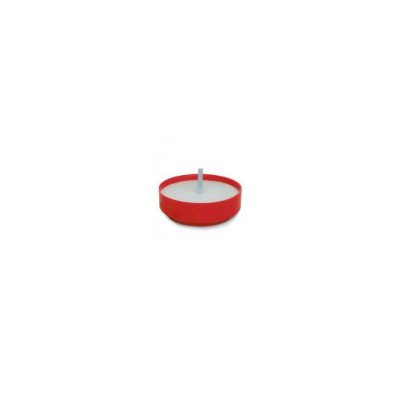The image depicts a very small, round red bowl, potentially about an inch or two in height, situated against a white background with no border. The bowl's contents appear to be a light grayish or tannish substance that reaches almost to its edge, suggesting it's in liquid form or possibly a thick wax. In the center of the bowl, there is a prominent stick-like object that could be a candle wick, a straw, or a spoon handle, standing resiliently upright. The bowl's shape is considerably flat compared to its height, and it is the only element in the image, with no shadow or additional context provided.